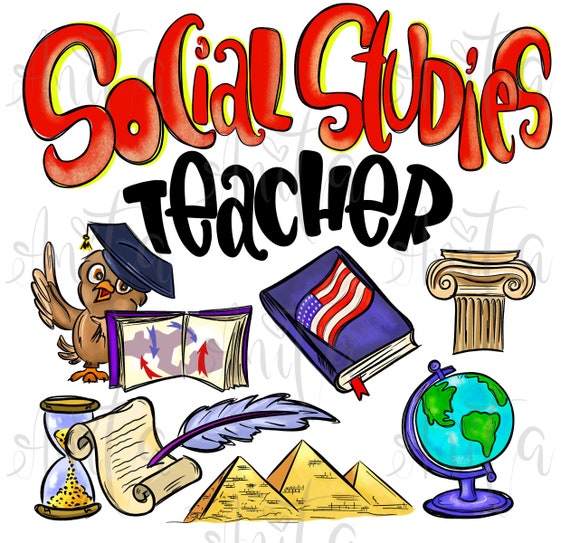The graphic at the top boldly displays the words "Social Studies" in an orangish-red color, followed by the word "Teacher" in black. Below the text, the image features a series of illustrative elements: starting on the left, a brown owl with a graduate hat tilted on its head has its right wing raised, as if in explanation. Next to the owl, an open book with arrows stands out. Below this is an hourglass with sand flowing through it. In the middle, a partially unrolled parchment with a feather pen rests beside three gold pyramids. To the right, a detailed globe with blue and green hues and a purple base sits prominently. Above the globe, the top of a pillar or podium is displayed, and to its left, another closed book bears an American flag on its cover. This array of images encapsulates various elements associated with the life and work of a Social Studies teacher.